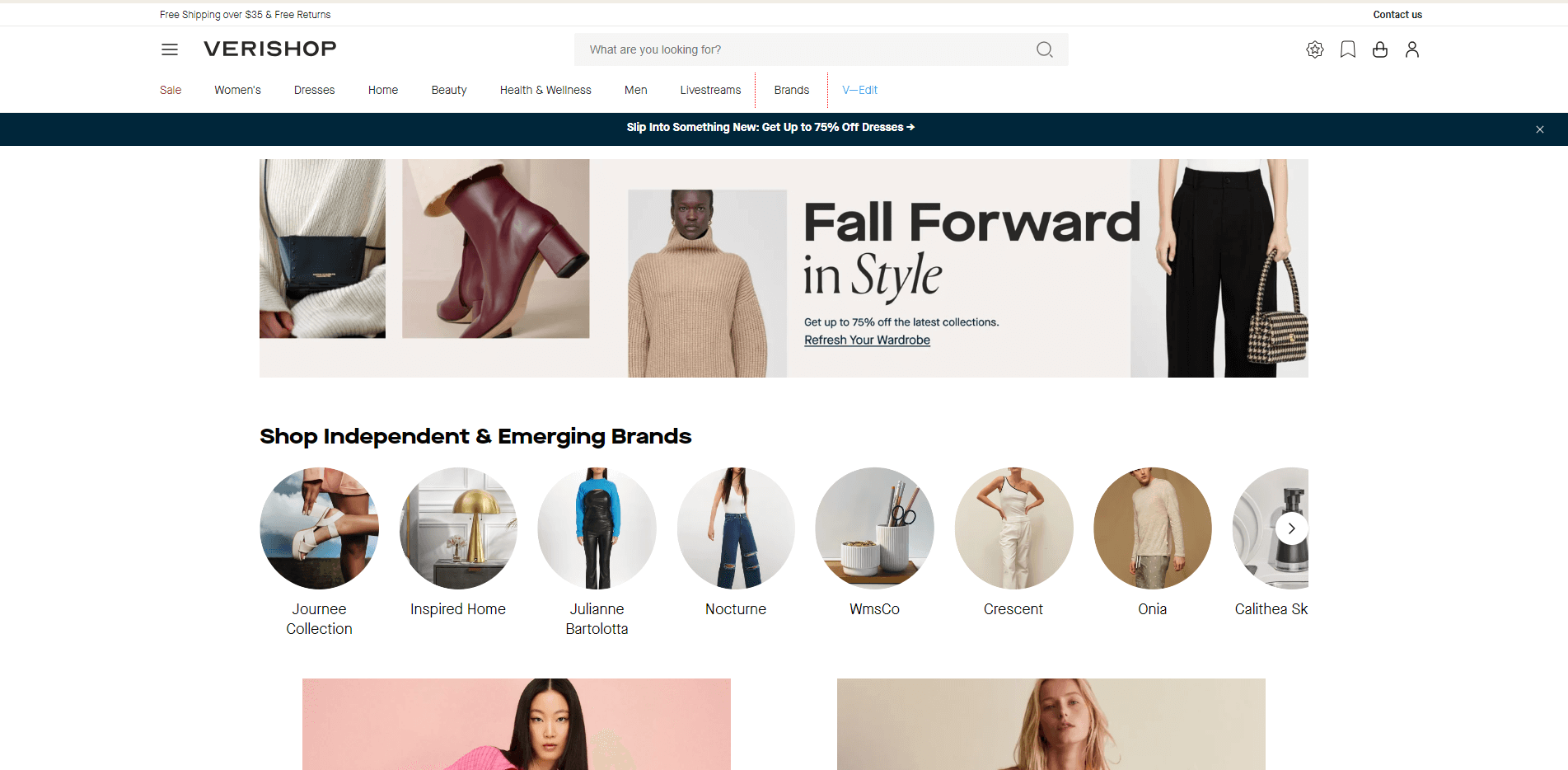In the screenshot of the webpage, the header is prominently displayed, reading "Very Sharp" and highlighting an offer of "Free shipping over $35" along with "Free returns." A search box invites users to "What are you looking for?" and next to it, there are a gear icon and a favorites icon. A generic default profile picture icon is also visible. Another tab labeled "Contact Us" is present along the top menu. 

The navigation menu lists various categories: "Sale," "Women," "Dresses," "Home," "Beauty," "Health and Wellness," "Men," "Livestream," "Brands," and "Edit." 

Below the navigation menu, there's a prominent black banner proclaiming "Something New," which advertises "Get up to 75% off dresses." The section beneath features images of a sweater, boots, another sweater, black pants, and a pocketbook. The accompanying text encourages shoppers to "Fall forward in style," promoting up to "75% off the latest collections" and urging them to "refresh your wardrobe."

Additionally, there is a call to "Shop independent and emerging brands," mentioning names such as "Journey Collection," "Inspired Home," and "Julianne Bartolotta."